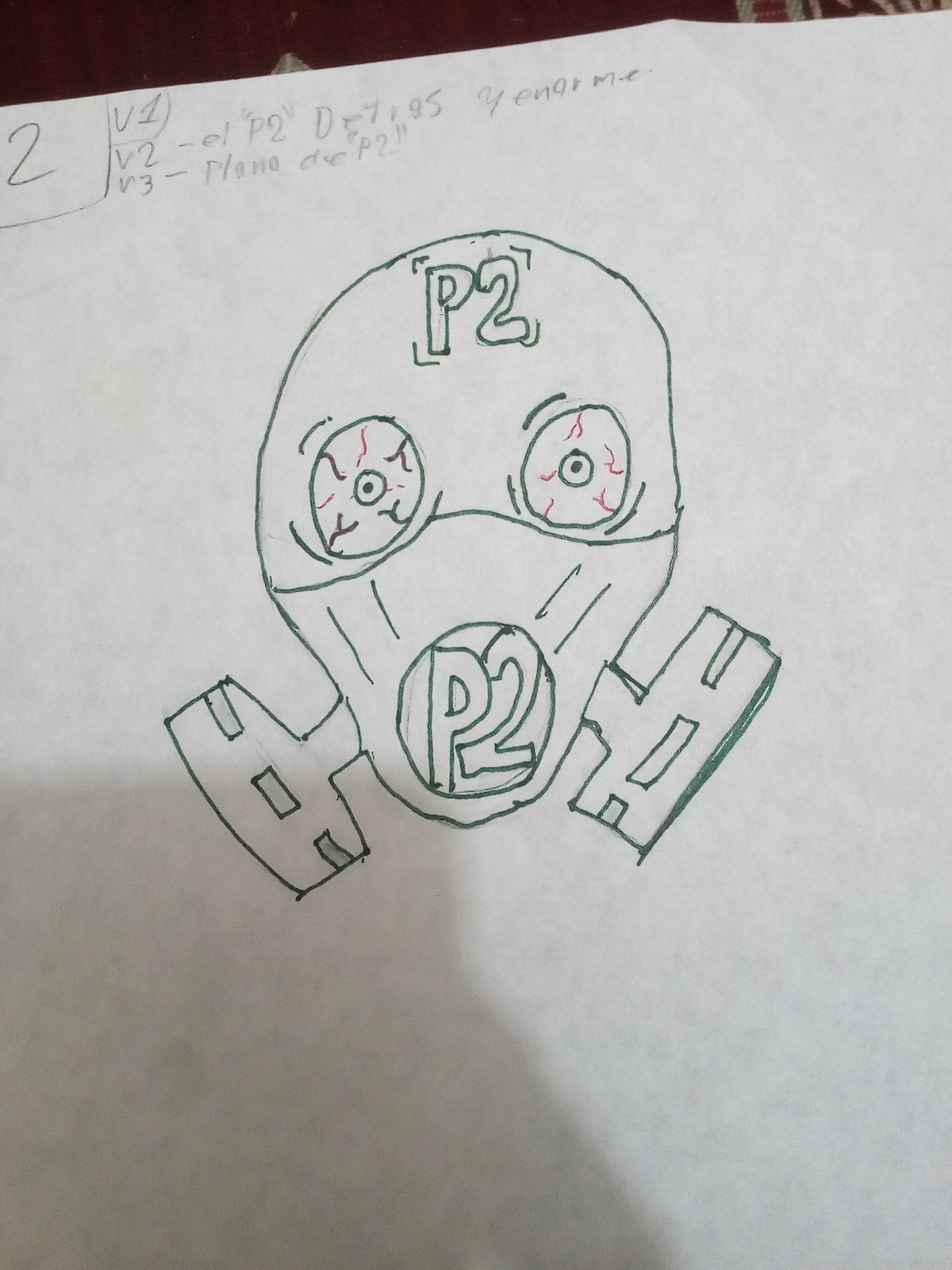The image is a photograph of a detailed drawing on a white piece of paper. At the very top of the paper, there is some indistinct writing, alongside the number 2. The primary focus of the image is a green pen drawing of a skeletal character wearing a gas mask. This gas mask, designed with intense precision, completely covers the face, including the nose. "P2" is inscribed on the forehead of the character, and again on the mouthpiece of the mask. The character has large, fear-filled eyes, which are enhanced with red lines to depict blood vessels, giving them a bloodshot appearance. The eyes are visible through the mask's holes and appear to convey a stark, unsettling emotion. Two air filters extending from each side of the mask further enhance its detailed representation, evoking a sense of desperate need for protection.